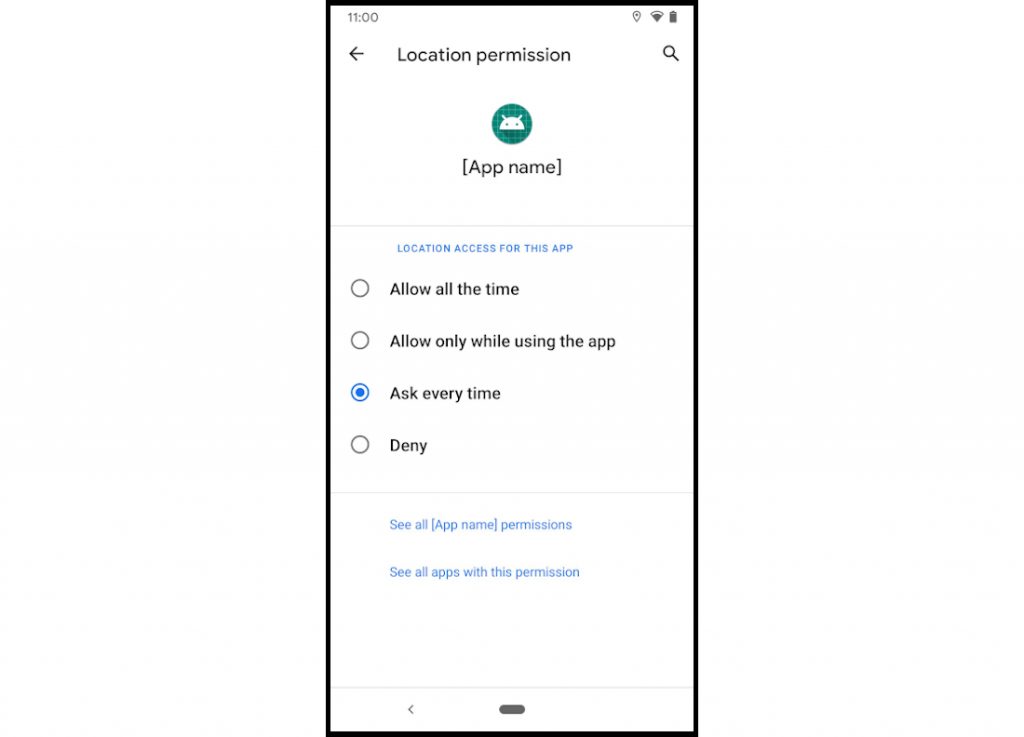A screenshot with a white background displays various elements at 11 o'clock in the time area. The interface includes icons such as a left-pointing arrow and a magnifying glass. Prominently, there is a green circle featuring the Reddit mascot face. Surrounding this central icon are various details:

- There are four radio buttons labeled: "Allow all the time," "Allow only while using the app," "Ask every time" (which is shaded in blue), and an option emphasizing in blue text, "See all" within brackets, along with "App name permissions" and "See all apps with this permission."
- The app name appears above "Location access for this app" which is highlighted in blue.
- At the bottom of the screenshot, there's a white rectangle with a left arrow, and in the middle of the bottom edge, there's an oval shape.

This detailed description captures the essence of what is displayed in the screenshot.